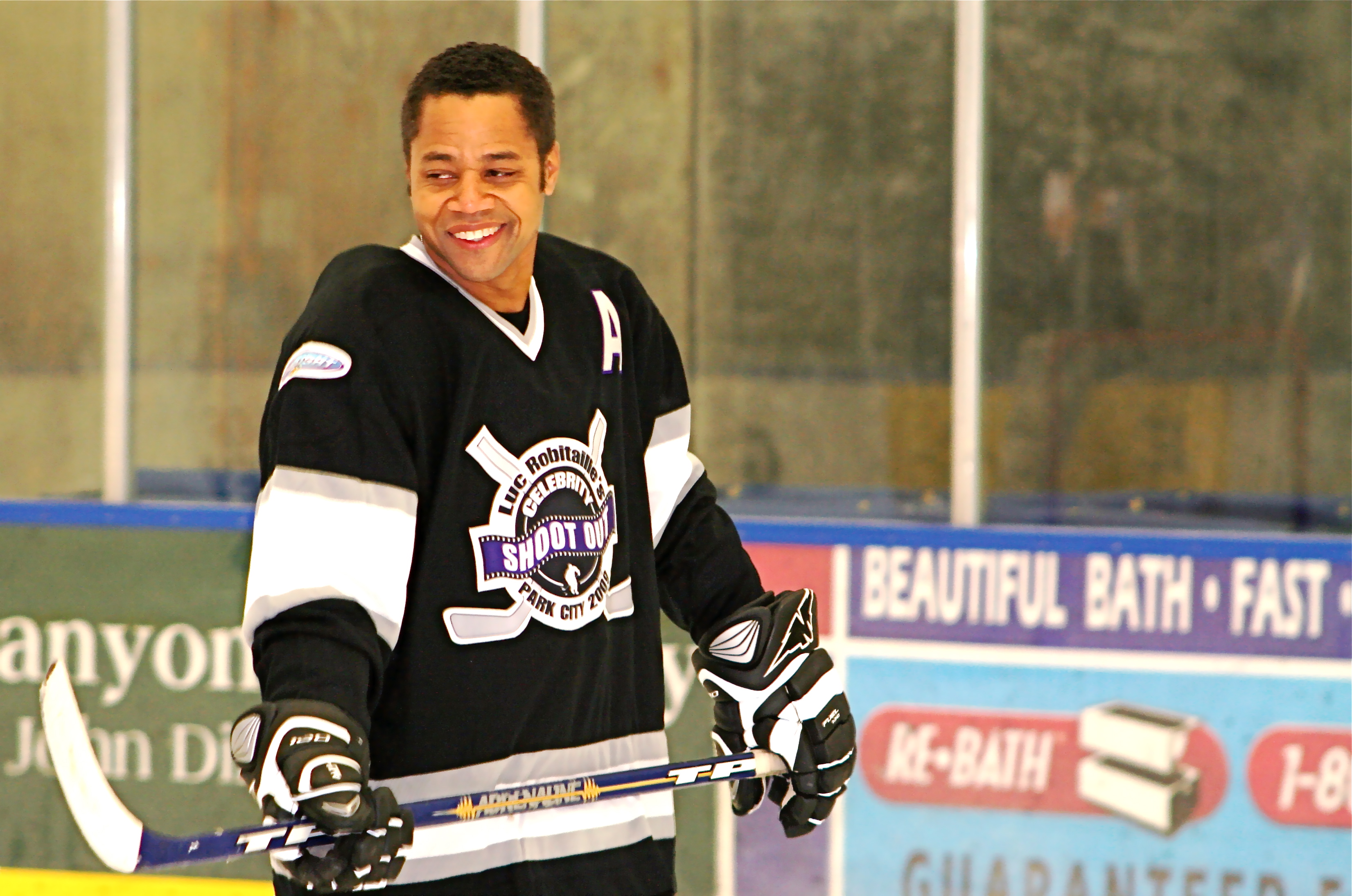In this detailed image, Cuba Gooding Jr. is captured in action at a hockey rink during a celebrity shootout event. He sports a black and white jersey with the words "Celebrity Shootout, Park City" emblazoned on the front. Complementing his attire, he wears matching black and white hockey gloves and grips a striking purple, white, and yellow hockey stick at waist level. Cuba is caught in a moment of joy, flashing a wide smile with visible teeth as he looks off to the left. The backdrop features a clear glass wall atop a barrier adorned with various advertisements, including phrases like "beautiful," "bath," and "fast." Although a patch is seen on his arm, it is too small to read. The scene vividly portrays the excitement and engagement of a celebrity event dedicated to the sport.